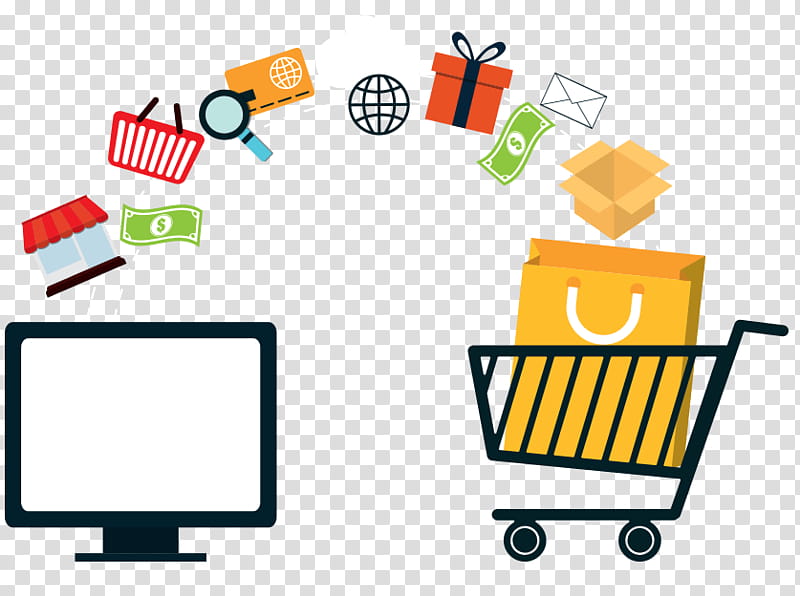The image depicts a black and white icon of a computer monitor on the left side, set against a background of small white and gray checkerboard squares. There's a simplistic black outline of a shopping cart on the right side with a yellow shopping bag inside it, featuring a white U-shaped handle. Above the shopping cart, curving towards the computer monitor, are various icons symbolizing online shopping. These include a green dollar bill, a magnifying glass, a white envelope, a beige cardboard box, an orange present with navy blue ribbon, an orange credit card with a white globe, a storefront, another green dollar bill, a red shopping cart, and a globe icon. The overall visual suggests the concept of items moving from online purchase via the computer into a shopping cart, representing the process of e-commerce.